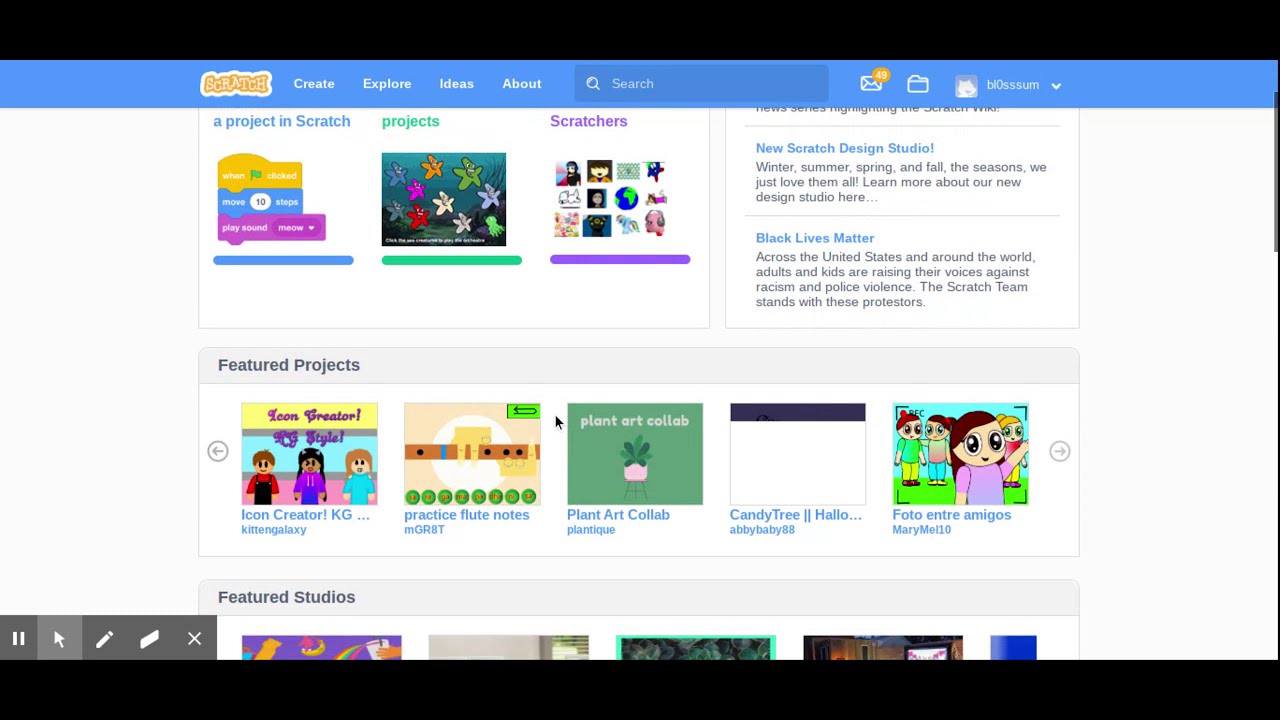### Detailed Website Screenshot Description

The screenshot features a web page from a website with a predominantly blue and white color scheme. Here's a breakdown of the elements:

1. **Header Section:**
   - **Top Left Corner:** The logo "Scratch" is prominently displayed.
   - **Navigation Menu:** Positioned to the right of the logo, there are four categories in white text: "Create," "Explore," "Ideas," and "About."
   - **Search Bar:** Located to the right of these categories.
   - **User Icons:** Further right, there's an email icon with the number 45 in orange, representing unread messages, followed by a folder icon, and then a profile icon. The background of this entire header section is blue.
   - **Top and Bottom Borders:** Both have a black background framing the site.

2. **Main Body:**
   - **Background:** The main content area is set against a white background.
   - **Top Section:** Features three categories listed horizontally: "Project and Search," "Projects," and "Scratchers."
   - **Right Sidebar:** Contains two sections: "New Scratch Design Studio" at the top and "Black Lives Matter" below it.

3. **Featured Content:**
   - **Section Header:** "Featured Projects" is prominently displayed in black text.
   - **Project Thumbnails:** Below this header, five different projects are displayed with blue text titles and corresponding thumbnails.
   
4. **Featured Studios:**
   - **Section Header:** "Featured Studios" is indicated, with the top portion of the section visible on the screen.
   - **Thumbnails:** Four studio images are partially visible within this category.

5. **Left Sidebar:**
   - **Icons:** A vertical gray rectangular background hosts several small icons:
     - A pause button
     - An arrow button
     - An edit button
     - A card button
     - An exit (X) button

This detailed depiction encapsulates the layout and design elements visible in the screenshot, providing a thorough understanding of the web page's structure and content.